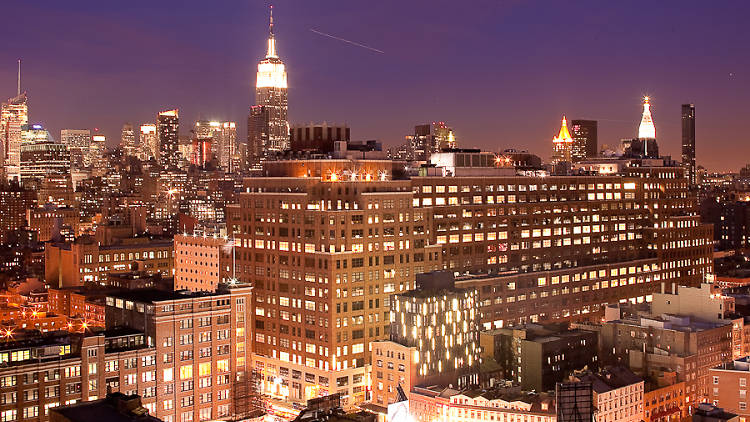The image depicts a vibrant city scene at dusk, dominated by a striking evening skyline. The sky features a gradient of dark purple hues with touches of pink and red near the horizon, transitioning to bluer tones as it reaches the top edge of the photo. The cityscape is filled with an array of buildings, varying in size and structure. In the foreground, two prominent brown buildings with numerous lit windows stand out; one is multi-story, rising approximately 12 to 14 stories tall, while the other is roughly half its height.

Behind these central buildings, a series of skyscrapers stretches left to right, their illuminated windows creating a dazzling display against the twilight sky. Notably, an especially tall building slightly left of center draws attention with its prominent spire reaching up towards the top of the image. To the right of this towering structure, a streak of light cuts diagonally downward through the sky, adding an intriguing element to the scene. Overall, the cityscape is bathed in the glow of countless lights, presenting a typical yet mesmerizing night view of a bustling city. Despite the intricate detailing of the architecture, the distance and scale offer no discernible presence of people, accentuating the grandeur and vastness of the urban environment.